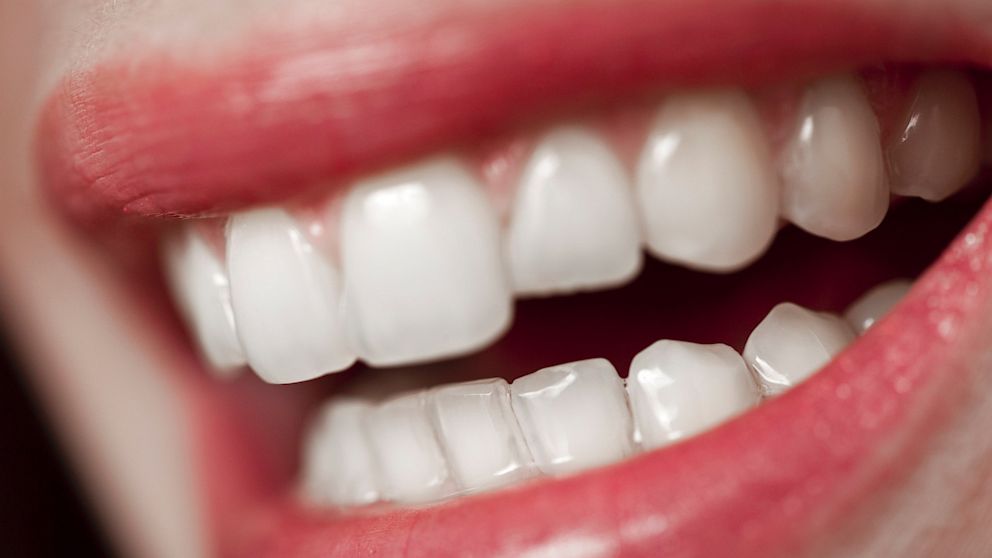The image is a very close-up shot of a Caucasian woman's mouth, open in a smile or laugh. Her extremely white, clean teeth are slightly apart, revealing straight, almost perfect alignment, possibly due to dental work like caps. Her gums are a healthy pink, and her bright red tongue is visible. Her lips, pulled tight in the act of smiling or laughing, are a natural pinkish-red, though possibly a bit dry. The skin around the mouth is fair, and the blurred background keeps all focus on her impeccable dental hygiene and vibrant smile.